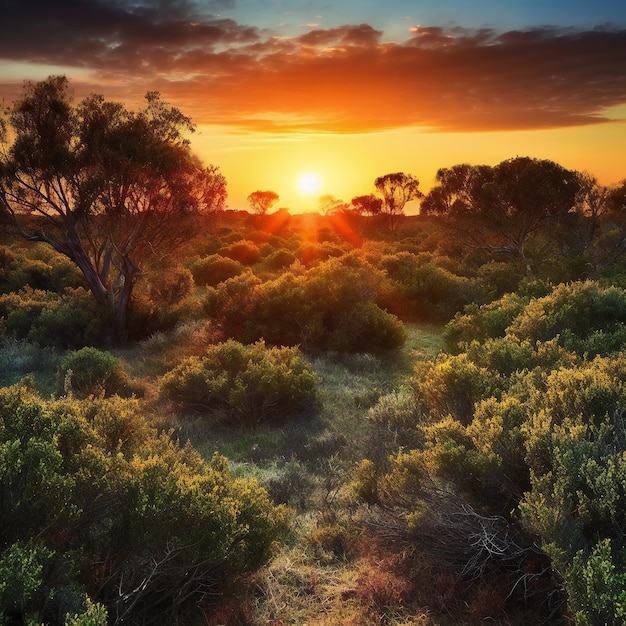This captivating image showcases a tranquil forest at either sunset or sunrise, with the sun sitting low on the horizon. The atmosphere is bathed in warm hues, transitioning from a vivid yellow near the horizon to a soft orange above, where a cloud catches the light and turns gray against a light blue sky. Dominating the landscape are numerous trees and dense patches of grass, undisturbed and thriving. A large tree with sparse leaves stands prominently on the left, mirrored by similarly sparse trees in the back right, while the rest of the foliage is thick and lush. The foliage near the camera in the foreground exhibits a mix of yellow, orange, and red tones, possibly illuminated by the sun's low angle. The ground appears dry, indicating a lack of recent rain, adding to the timeless, untouched quality of this serene natural scene.